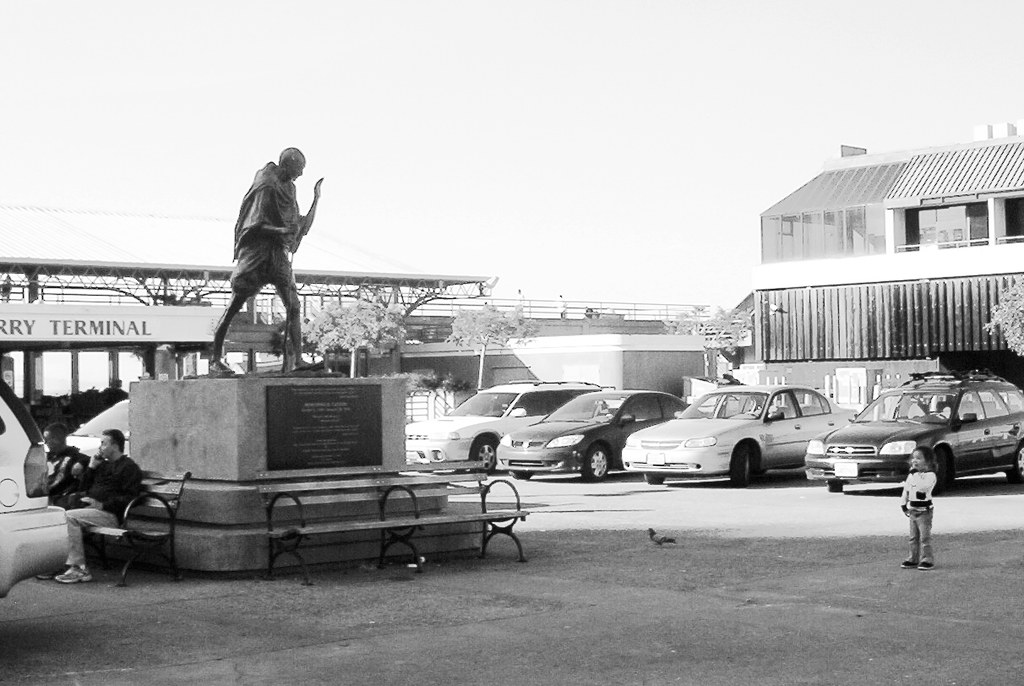In this black and white photograph, we see an outdoor setting in the middle of the day, centered around a historical statue that resembles Gandhi. The statue, positioned slightly left of center, stands atop a three-tiered granite base with a plaque on the front, though its text is unreadable. Gandhi appears to be in motion, with his left hand raised.

Surrounding the statue is a circular bench where a man in blue jeans and a black jersey sits to the left, while a young boy, around six or seven years old wearing a white shirt and brown pants, stands to the right. A pigeon is on the ground between the boy and the statue. 

Off to the left of the image, partially obscured but identifiable, is a ferry terminal. Only part of its sign, “RRY Terminal,” is visible. Behind the statue, there is a three-story building with distinctive features: an A-framed roof, a picture window, a small balcony on the uppermost floor, and a lower section of vertically striped wood paneling. Four cars—a black station wagon, a white sedan, a darker smaller car, and another white vehicle—are parked in front of this building. To the right, trees with leafy tops add to the scene. Despite its grayscale presentation, the photograph clearly captures a sunny day, with sunlight highlighting the parked cars and casting shadows that enhance the depth and detail of the composition.